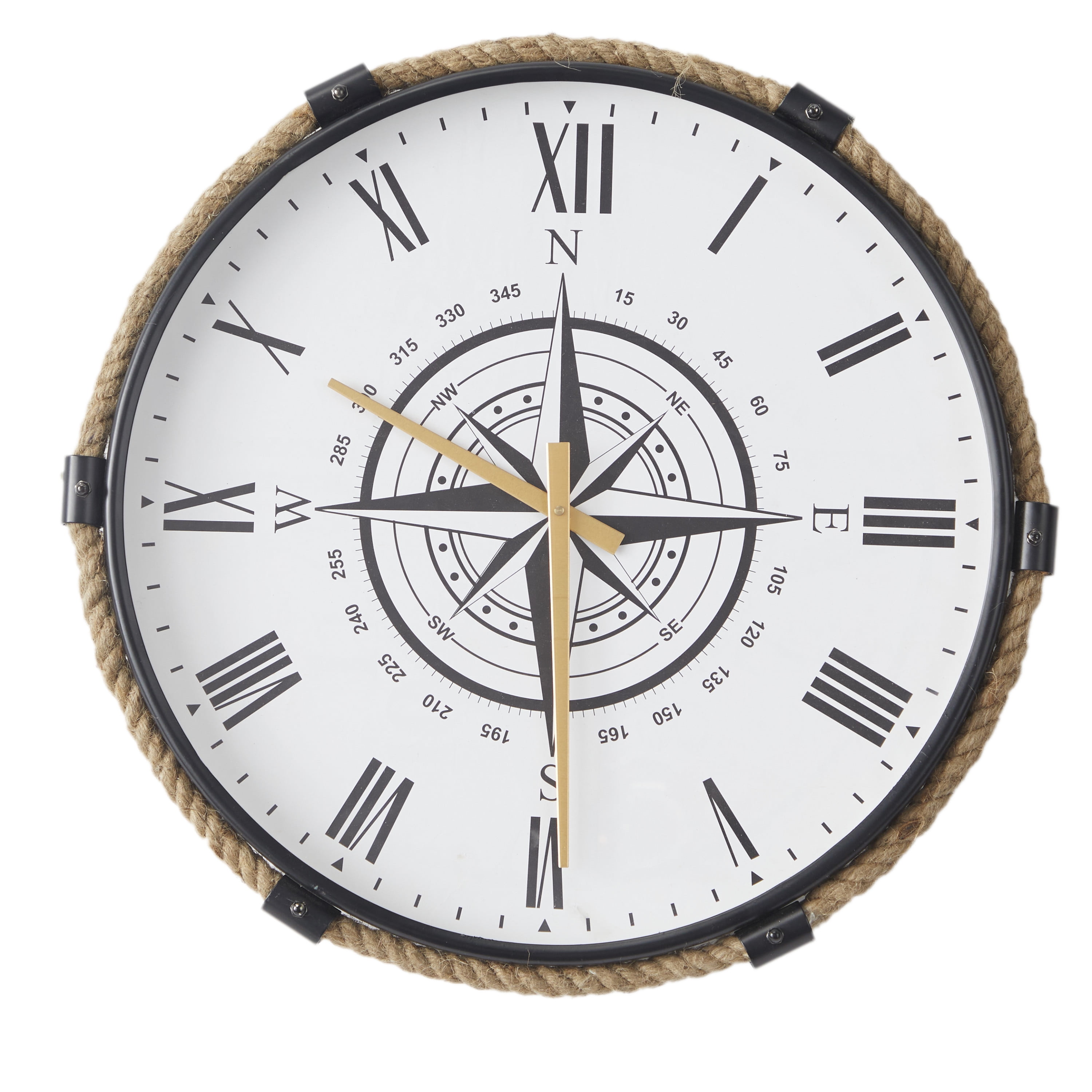This unique object is a combination of a compass and a clock, boasting a distinctive and artistic design. The circular device features a white face bordered by a tan brown twisted braid that encircles its entire circumference. Six small black clips secure the rope at the positions equivalent to 1, 3, 6, 7, 9, and 11 o'clock. The face of the device houses Roman numerals marking the clock hours, with capitalized lettering for each numeral. 

Within the clock's face lies a star-like structure with gold arms; one long gold hand points to the numeral VI for the hour, while a shorter gold hand indicates the minutes. Additionally, positioned among the Roman numerals are the cardinal directions (N, E, S, W), defining its functionality as a compass. The combination of the clock hands and compass points, set against the white background with Roman numerals, creates an intricate and multifaceted instrument that merges timekeeping with navigation.